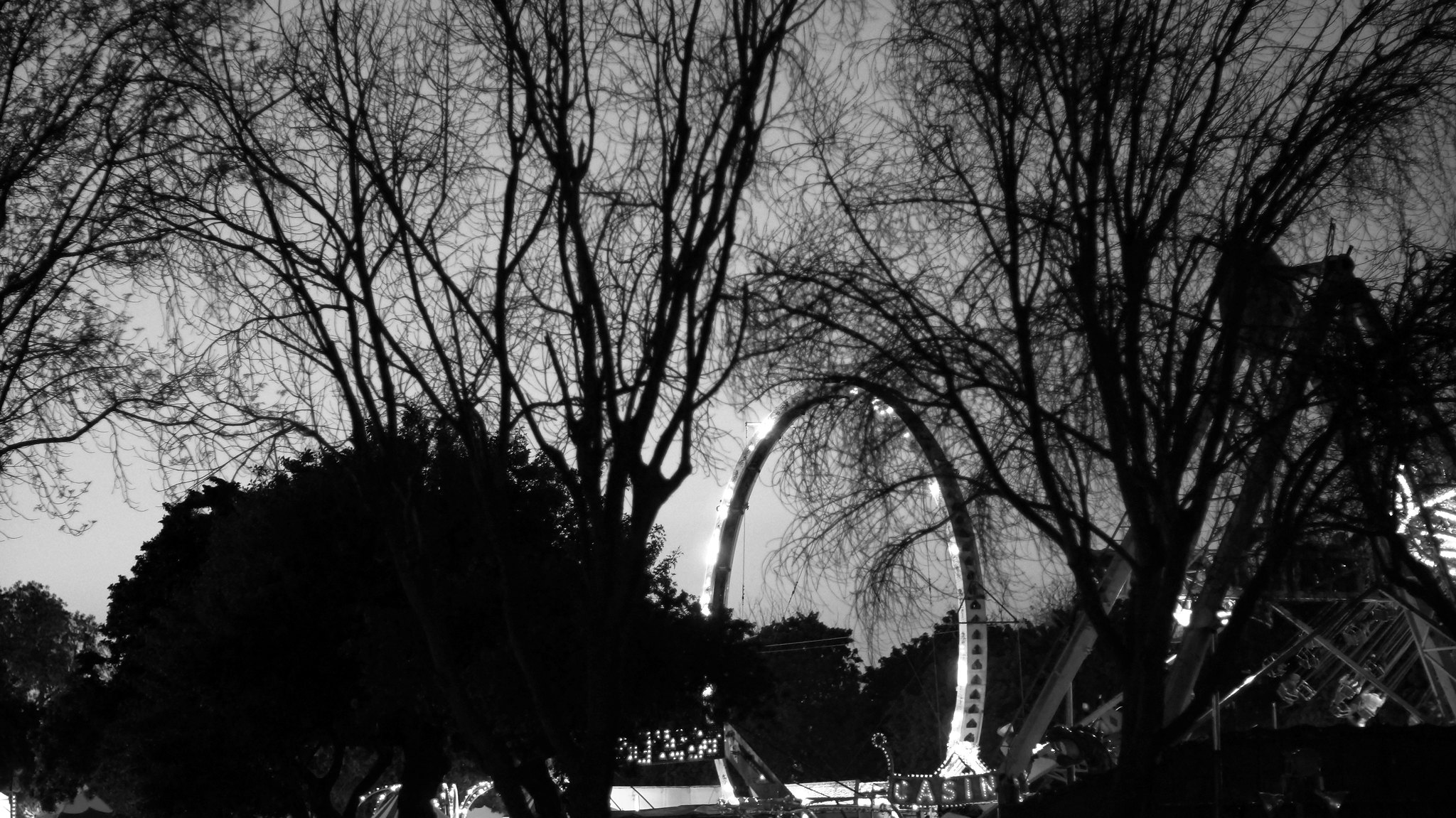This black-and-white photograph, rectangular in shape, captures an outdoor nighttime scene at what appears to be a carnival or amusement park. The sky, rendered in grayscale, gives a dull, ominous appearance, contrasting sharply with the brightly lit subjects in the image. Tall, mostly barren trees with scrawny tops frame the scene, their dark silhouettes dominating the background. In the center of the photograph stands a large, illuminated structure resembling a Ferris wheel or a similar ride, with a prominent circular shape adorned with lights along its exterior.

A lit-up archway beneath the wheel bears a partially visible banner spelling out "C-A-S-I-N," suggesting the word "casino." To the right, the image hints at another ride, possibly a roller coaster, with its lit archways and moving lights partially visible. On the left, additional lit areas peek through the dense foliage, indicating more carnival attractions just out of full view. The overall ambiance is very dark, with the trees and shrubbery almost blending into the night, casting a mysterious and somewhat eerie tone over the entire scene.